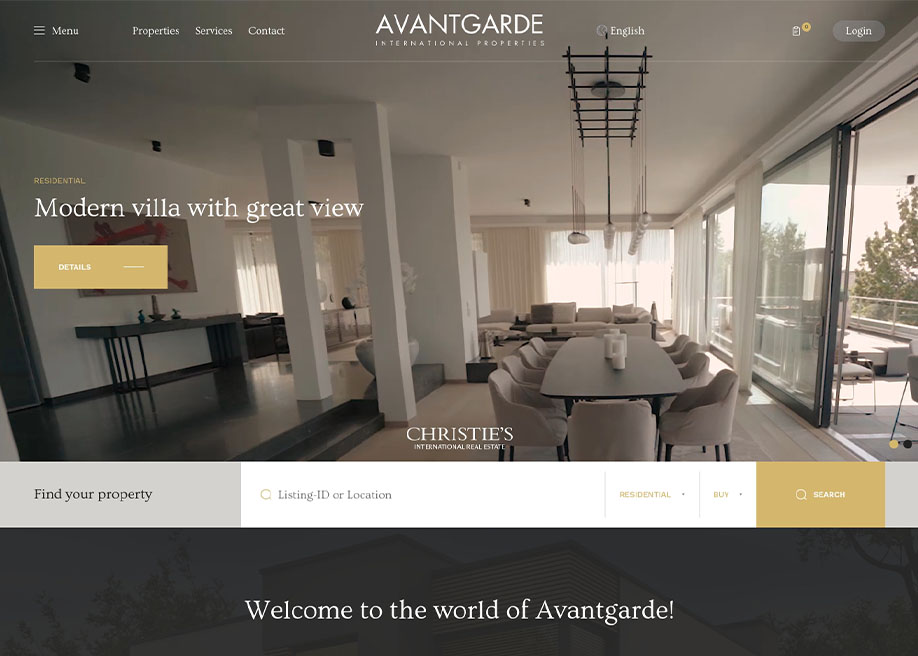**Image Caption:**

A screenshot of a luxurious real estate website is presented, featuring a lavish dining room as the background. The dining room boasts clean wooden floors and a pristine white dining table, complemented by an elegant white ceiling. Stylish lights hang over the dining table from strings attached to a black rack. Architectural columns separate this area from a raised section, and large open windows reveal an elevated porch bathed in sunlight, emphasizing the opulence of the space.

At the top center of the webpage, "Avant-Garde International Properties" is prominently displayed. To the right, the interface indicates English as the selected language, accompanied by a small, unclear icon and a login button. On the left, navigation links include Contact, Services, Properties, and Menu.

The focal point of the webpage features the text "Residential Modern Villa with Great View" slightly off-center to the left, accompanied by a tan 'Details' button. At the bottom center, the logo "Christie's International Real Estate" is visible, followed by a gray 'Find Your Property' button, a search field labeled 'Listing ID or Location,' and dropdown menus for 'Residential' and 'Buy.' A tan orange 'Search' button is placed beside these elements. 

Below this is a black banner with the text "Welcome to the World of Avant-Garde," set against a faint roofline in the background.